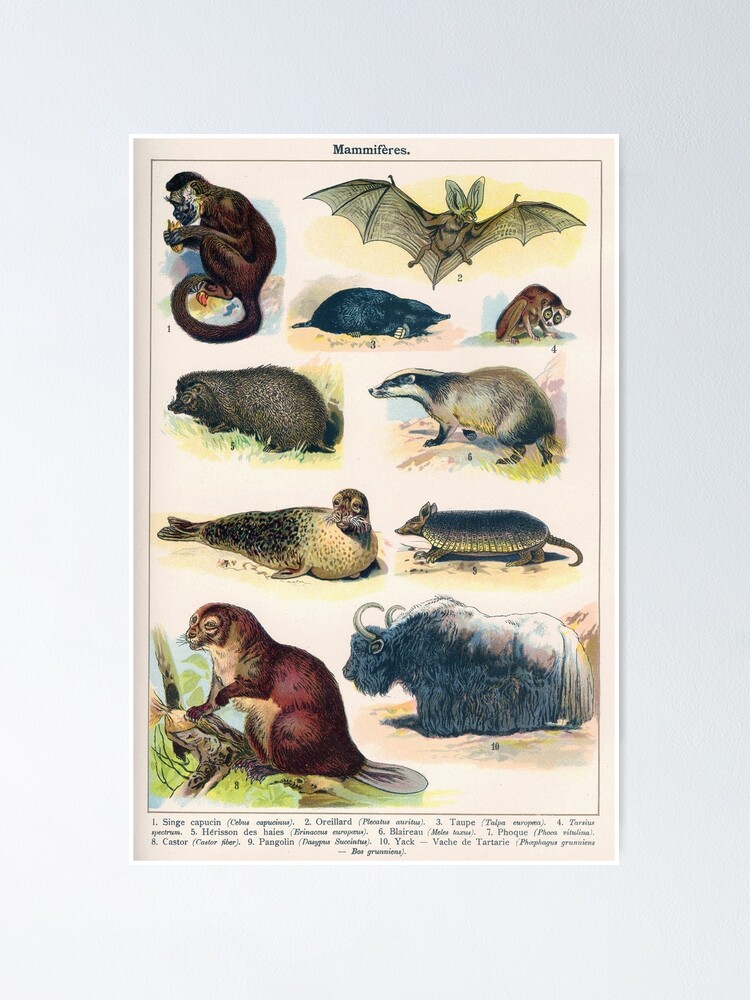This detailed poster features an educational collection of various mammals, likely from an educational book or museum display. It has a light cream or slightly pink background with the title "Mammiferes" printed in small capital letters at the top. The animals are illustrated in an old-style drawing, filled with dark colors, and each is numbered with corresponding labels at the bottom. Among the distinct creatures depicted are:

1. Singe Capuchin (Pallas Cephcebus capsinus) - a capuchin monkey in the top left.
2. Oriola (Placendis oritis) - an oriole.
3. Taupe (Talpa europes) - a toad.
4. Tarsius Spectrum - a tarsier, possibly hard to read.
5. Harrison Desmus (Erinaceus europaeus) - a hedgehog.
6. Blereau (Blarina tessius) - a mole.
7. Popti (Potorous retulina) - a potoroo.
8. Castor (Castor fiber) - a beaver.
9. Pangolin (Deriperes succinctus) - a pangolin.
10. Yak (Vashni tartari) - a yak.

Some additional animals include a war buffalo with horns, likely a boss guenonis, an armadillo, a lemur-like creature, and a bat. The illustrations also show a seal with white and gray coloring at the bottom. Each creature is meticulously depicted to provide an educational overview of their variety and characteristics.